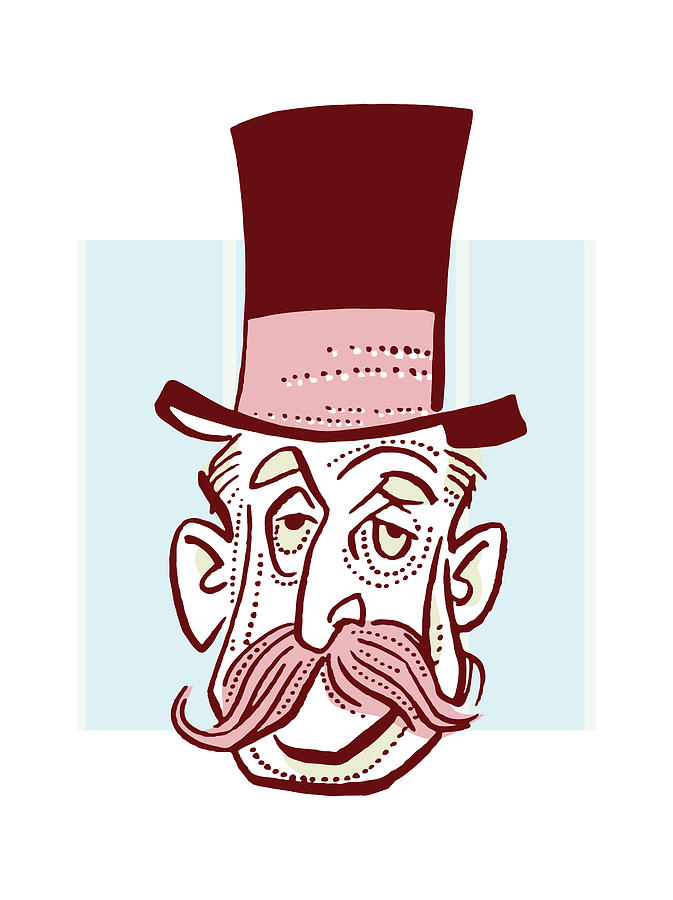The image is a cartoonish portrayal of a gentleman wearing a tall, maroon-colored top hat with a light pink band featuring maroon dots. His face is detailed with a prominent pink handlebar mustache speckled with maroon dots, a long nose, large ears sticking out, and half-closed, bored-looking eyes. The gentleman's white skin is accented with maroon dots on his forehead, under his eyes, cheeks, and chin, giving his appearance a stippled texture. His expression suggests boredom or disengagement. The background is a soft baby blue square, providing a gentle contrast to the man's detailed, colorful visage. The artwork focuses solely on his head and hat, omitting any neck or shoulders.